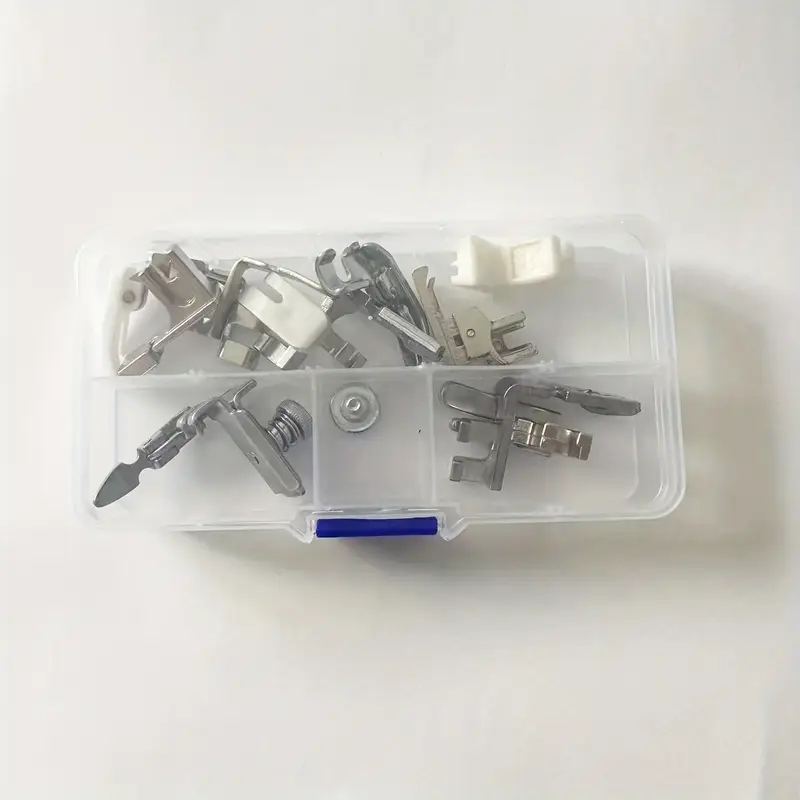The image depicts an aerial view of a clear plastic organizer used for storing various small tool parts. The organizer has a transparent body with an opaque but colorless appearance, and a distinct blue handle at the front. Inside the organizer, there are four compartments: one large section at the back and three smaller ones in the front. Each compartment is filled with an assortment of metal and plastic parts, predominantly silver in color.

The contents include numerous screws, clamps, shelf mounting brackets, and potentially drawer mounting accessories. There's also one notable white plastic shelf mounting bracket amidst the otherwise metallic collection. While the specific purpose of every item isn’t entirely clear, the pieces appear to be related to construction or repair tasks, possibly for things like door frames, faucets, or similar hardware applications. The general use case suggested for these parts includes activities like attaching fixtures or mounting shelves. The background of the image is white, which helps to highlight the contents of the organizer.